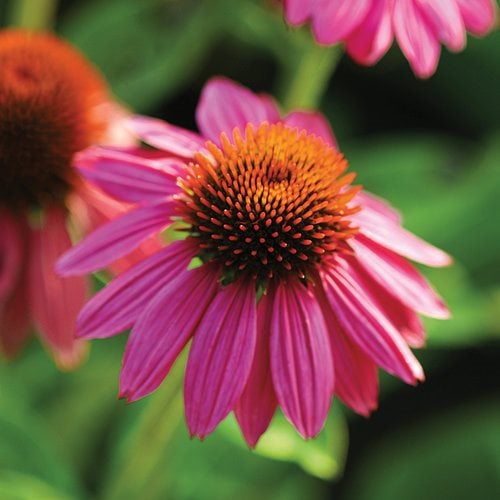This image captures a close-up of a vibrant pink flower, likely a daisy, positioned prominently in the center. The main flower showcases multiple layers of long, slender petals exhibiting slight ripples. The petals extend outward at a downward angle, encircling the flower in a harmonious pattern. At the heart of the flower, an orange bulbous center draws attention with rows of tiny orange spikes emerging from a blackish background, creating a plush, textured appearance. Green elements peek through at the base of the central bulb, subtly contrasting with the vivid petals. The blurred background, indicative of outdoor surroundings, features indistinct green leaves and hints at the presence of more flowers of the same kind. Notably, partial views of additional flowers appear at the upper right and left edges of the frame, one showing some pink petals and the other revealing a hint of another bulbous center and petals. The photograph, a square three-inch by three-inch frame, delivers a striking and detailed portrayal of this captivating pink flower amidst a natural, though unfocused, backdrop.